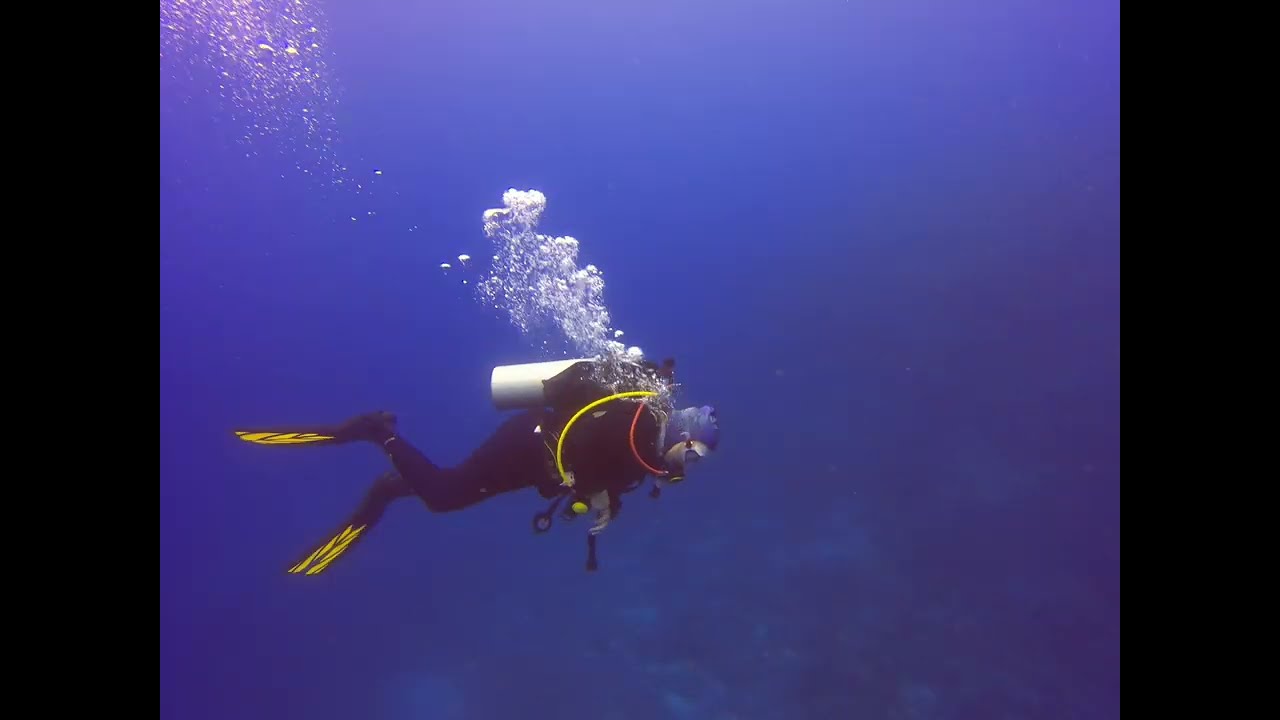In this vivid underwater scene, a scuba diver, dressed in a black wetsuit with red and yellow accents, navigates through a deep blue ocean. Positioned in the bottom left of the image, the diver appears horizontal, looking downwards, possibly examining the ocean floor or the sparse, blurry coral reefs that are barely visible amidst the shades of blue water, which shift to a hint of purple closer to the surface. The diver is equipped with black and yellow flippers, a blue and silver mask, gloves, and a snug headpiece. An oxygen tank, gray in color, is strapped to his back, with several colored hoses connecting the tank to his mask. Bubbles, white and clear, trail behind him, rising up towards the surface, adding a dynamic sense of movement to the scene. The image is framed with a black border on the left and right sides, accentuating the vibrant underwater hues and emphasizing the diver as the main focus of this serene and captivating aquatic snapshot.